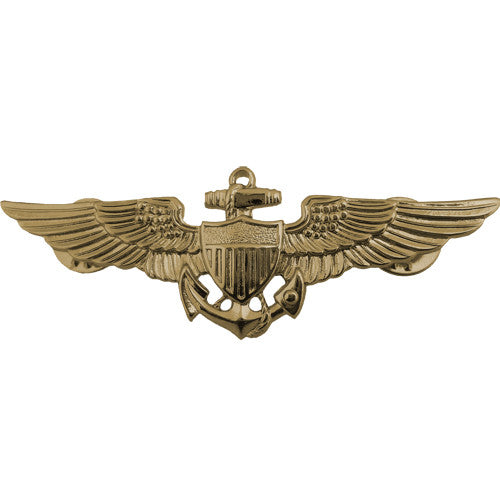This image showcases a detailed insignia resembling the wings that airlines use in their branding, though it specifically represents naval aviator wings. The entire piece is crafted in a bronzy gold color, evoking the appearance of medals or pins worn by pilots on their uniforms. The wings span outward with intricate, horizontal lines across their surface, signifying meticulous design. 

At the heart of the wings, there is a prominent anchor. This anchor is crafted in a shiny, bright gold and is central to the composition, symbolizing a connection to naval tradition. Within the anchor, there is a shield, which enhances the emblem's sense of prestige and valor. Some descriptions note that the shield appears to have bars or a cross-like design, adding layers of symbolism that suggest protection and honor. The overall imagery is emblematic of achievement and service, reminiscent of the pins worn by naval aviators upon their graduation from flight school.